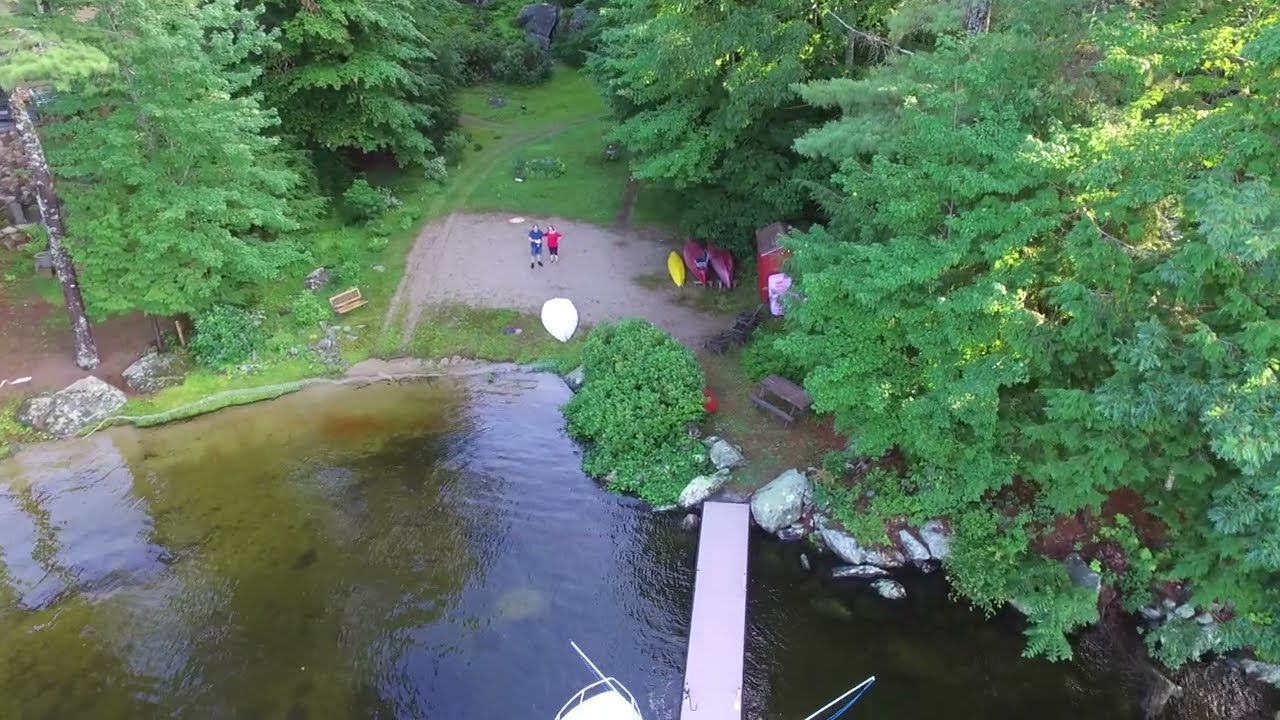This is a high-angle drone shot capturing a tranquil lake in a lush, forested area that appears to be a well-equipped campsite. The clear, brownish water of the lake reveals rocks and large boulders beneath the surface, suggesting it's not very deep. A wooden pier extends into the lake, from which a boat is moored. Below, there is a gravelly area where a man in a blue shirt and a woman in pink stand, possibly controlling the drone. Nearby, a pile of kayaks lies on the ground next to a small red shed that resembles an outhouse. The campsite features tall trees, a path leading to the lake, and a bench near the dock for boat unloading. It is an inviting scene, ideal for camping and water activities.